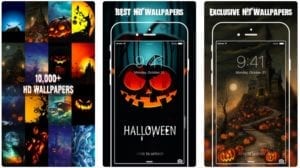The image features three small rectangular screens, all identical in size, displayed in a row. Each screen showcases a different set of HD wallpapers with a Halloween theme. 

The first screen on the left advertises "10,000+ HD Wallpapers" with a variety of spooky Halloween images. The preview shows a dark, eerie collection including a haunted stump and several jack-o-lanterns, arranged within a grid of 16 images. The overall aesthetic is quite dark and atmospheric, clearly designed to evoke a sense of Halloween spookiness.

The middle screen is labeled "Best HD Wallpapers" and features an outline resembling a phone. Inside this outline, a particularly menacing jack-o-lantern with glowing red eyes and an orange nose and mouth fills the screen. Above this menacing face, the word "Halloween" is written in a festive, stylized font. The background of this wallpaper is a deep blue, with silhouettes of trees adding to the eerie ambiance.

The screen on the far right displays "Exclusive HD Wallpapers," again within a phone-shaped outline. This preview showcases an intricate scene of a haunted mansion bathed in shadow. A large, low-hanging moon illuminates the left side of the scene, casting an ominous glow over a twisted tree and a winding path that leads up to the mansion. Along the path, several jack-o-lanterns with varying expressions light the way, creating an unsettling yet captivating visual composition.

Overall, each screen effectively contributes to a cohesive theme of dark, spooky, and immersive Halloween imagery.